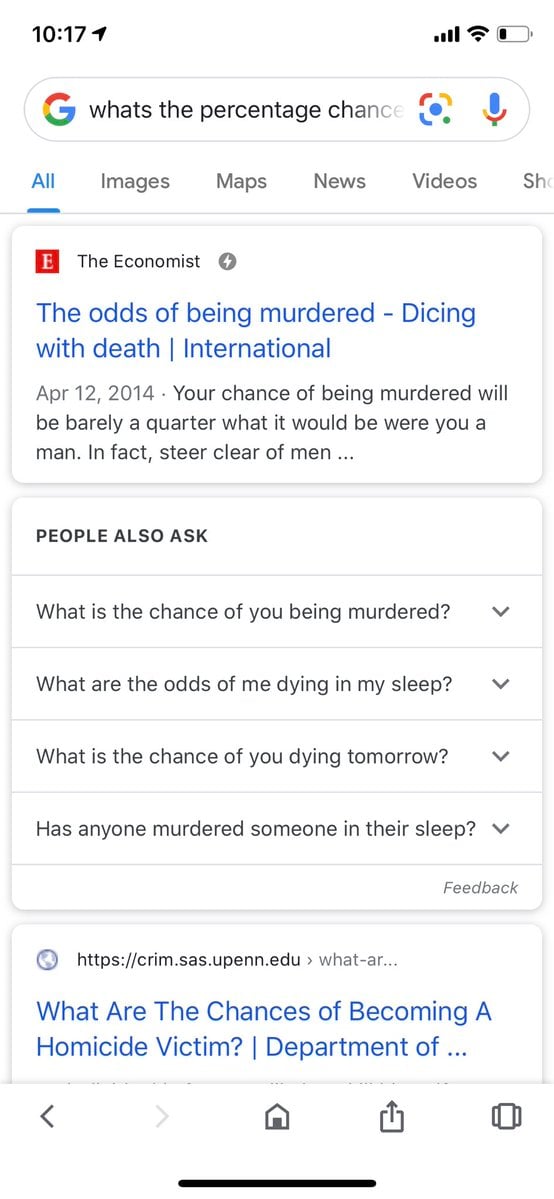The image displays a Google search results page on a mobile device, captured at 10:17 AM. The page has a large white search bar at the top, featuring the question "What's the percentage chance?" beside the multicolored Google logo and microphone icon. The phone's battery life is critically low, but the device has a good internet connection, as indicated by the blue highlighted and underlined signal icon.

Below the search bar, the first search result is from The Economist and discusses the odds of being murdered, noting that the chance of being murdered is significantly lower for women compared to men. The snippet abruptly ends mid-sentence. Other related queries by users include questions like "What is the chance of you being murdered?" and "What are the odds of me dying in my sleep?". Additional results mention the chances of becoming a homicide victim, but the text gets truncated.

At the bottom of the phone screen are navigational icons including the home button, download button, and several arrows, indicating this is a screenshot of an active internet search session on a mobile device.